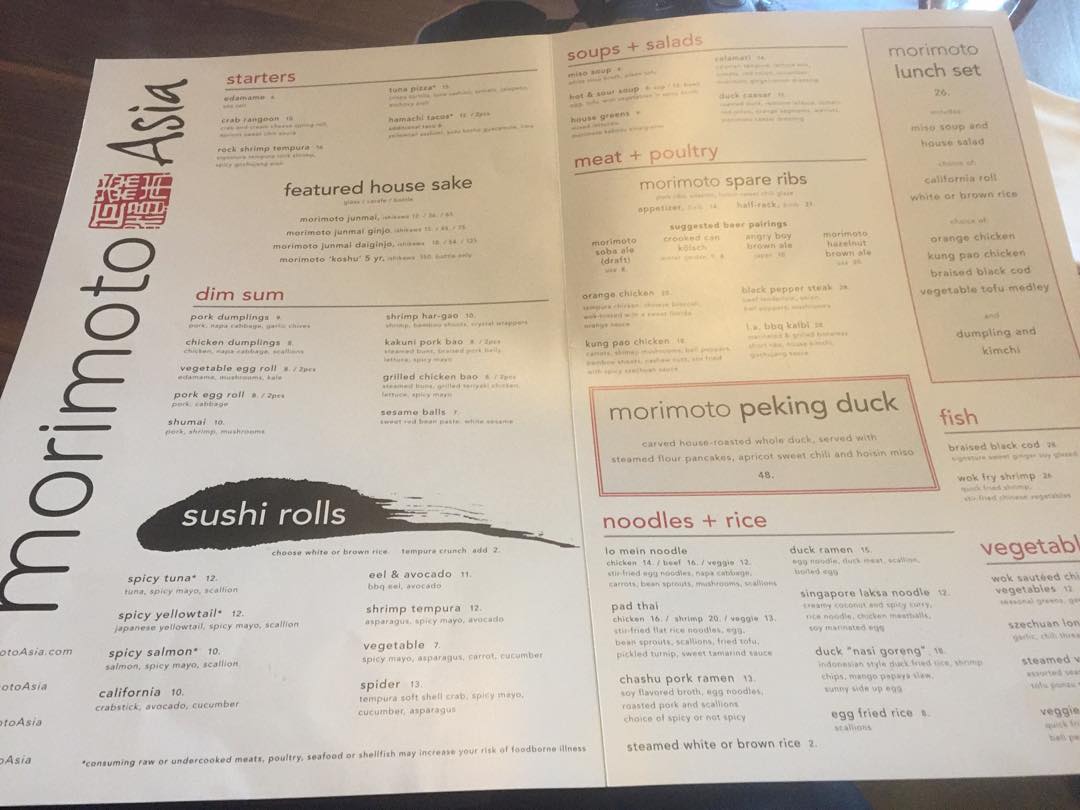This photograph captures an open menu resting on what appears to be a brown wooden table. The menu, printed on white paper, is laid out across two pages divided by a vertical line. The design and content of the menu are described as follows:

**Right Page:**
The header features the word "Morimoto" along the side, accompanied by a traditional Japanese stamp graphic, adjacent to the word "Asia." At the top of this page, the section labeled "Starters" lists six items, too small to discern. Beneath this, the "Featured House Sake" section includes four drink options, also too small to read. Following this, the "Dim Sum" section lists eight items, their details remaining indistinct. Below a prominent black smear, the "Sushi Rolls" section is highlighted in white font, offering eight rolls, their specifics unreadable.

**Left Page:**
This page's topmost section titled "Soups and Salads" is underlined in black, followed by a list of five indistinct items. The next section, "Meat and Poultry," introduces the "Morimoto Spare Ribs" with two lines of smaller, illegible text, followed by an additional eight items. A notable gray square highlights the "Morimoto Peking Duck" dish. The final section titled "Noodles and Rice" presents another set of eight items that are too small to be read.

The layout and minor details, such as the graphical elements and section headers, provide a structured overview despite the small text making individual menu items indistinguishable.